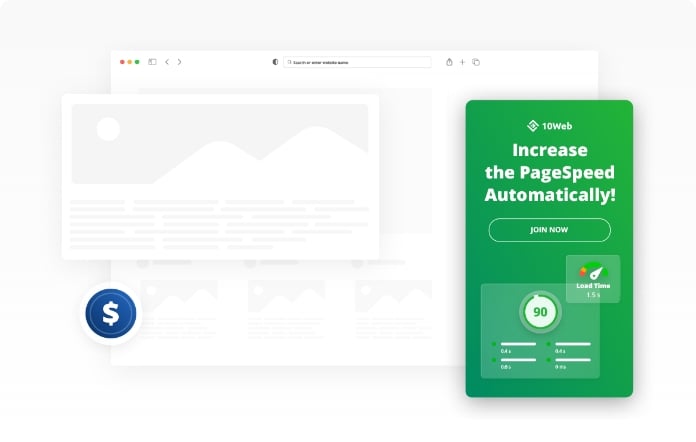The image depicts a website with a cluttered interface containing small and difficult-to-read text. Dominating the right side of the screen, there is a pop-up box promoting an automatic page speed increase service, prompting users to "Join Now" through a prominently designed button shaped like a hybrid circular-rectangular form. At the very top of the screen, the page banner displays "10Web" accompanied by a logo on its left side. Below this, there is an indicator for the page speed, which is encircled by the numeral 90, further dissected into four categories. Unfortunately, due to the small font size, these categories are largely indiscernible. Additionally, there is a white text box indicating the load time in seconds, partially overlapped by the 90-page speed marker. The overall layout is defined by a combination of white typography and various geometric elements positioned mostly on the right-hand side of the interface.